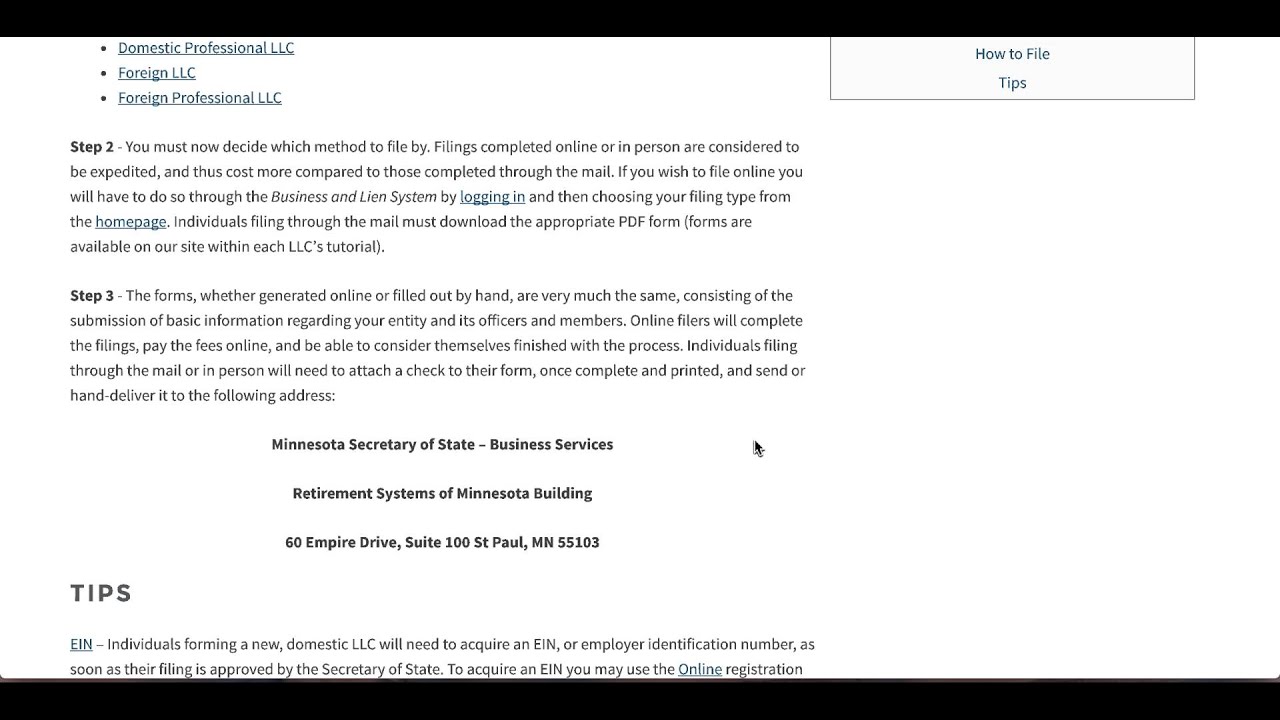A screenshot captures a step-by-step guide for filing Limited Liability Company (LLC) forms. At the top of the image, a prominent black bar features the page title. Below it, blue text lists various LLC types: Domestic Professional LLC, Foreign LLC, and Foreign Professional LLC. 

**Step 1:** The viewer is directed to decide on a filing method. The guide explains that online or in-person filings are expedited and therefore more expensive than mail-in filings. To file online, users must log in to the Business and Lien System and select their filing type from the homepage. For mail-in filings, individuals must download the appropriate PDF form available on the website's new LLC tutorial section. 

**Step 2:** Whether filing online or by mail, the forms require the same basic information about the entity, including details about its offices and members. Online filers complete the forms, pay the fees online, and finish the process digitally. Mail or in-person filers must attach a check to the completed forms before mailing or hand-delivering them to the following address: 
Minnesota Secretary of State, Business Services, Retirement Assistance, Minnesota Building, 60 Empire Drive, Suite 100, State Hall, MNS55103.

**Step 3:** Filers forming a new Domestic LLC must acquire an Employer Identification Number (EIN) as soon as their filing is approved by the Secretary of State. The guide concludes by noting that obtaining an EIN involves online registration.